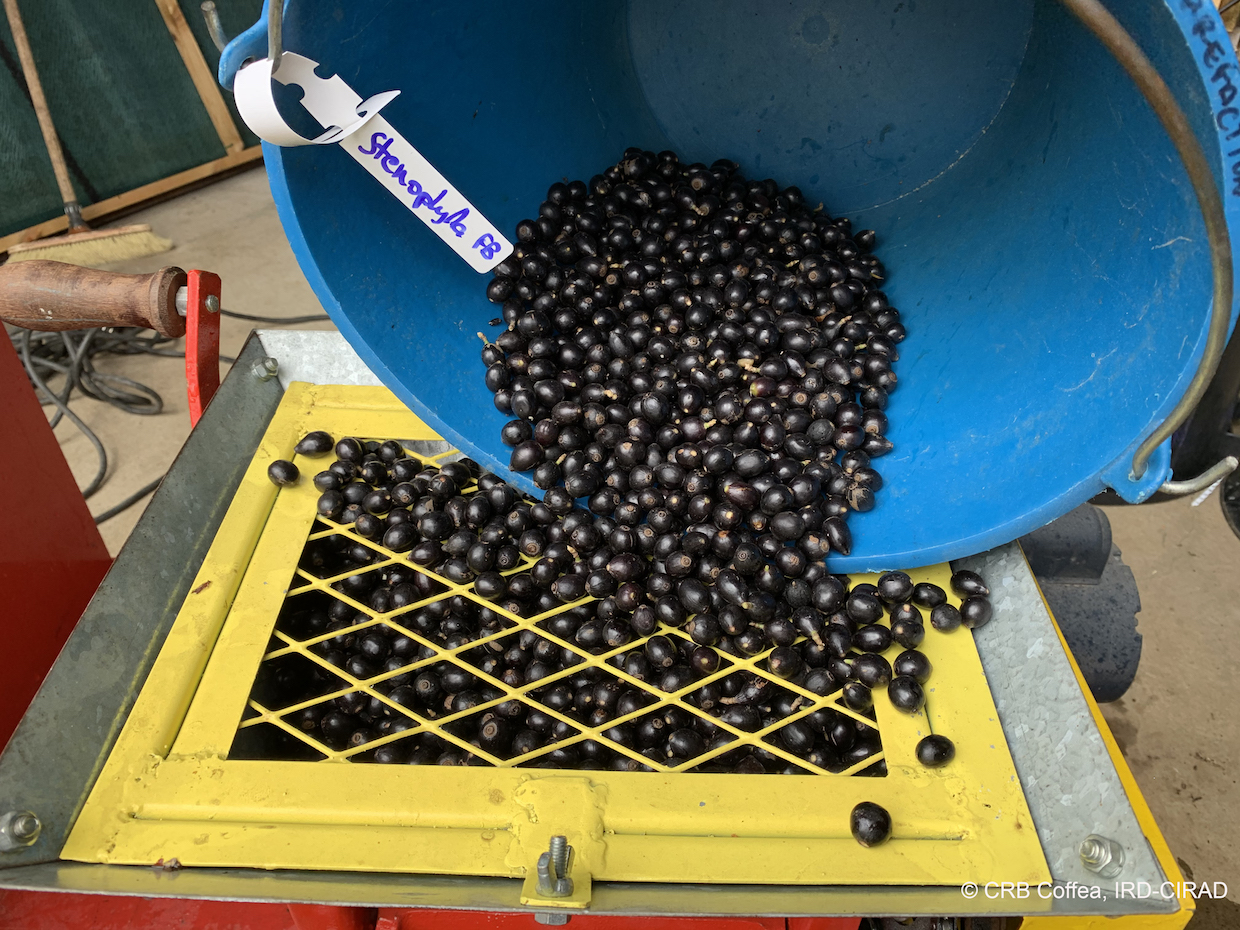This close-up, outdoor photograph captures a blue bucket filled with what appears to be Stenophylla beans, also labeled as "Stenoplida FB," being poured into a machine at a coffee processing facility. A bright yellow screen covers the opening of this hopper or grinder, filtering the beans while preventing the bucket from falling through. The handle attached to a red arm on the left-hand side suggests that this might be a manual grinder. The yellow screen is overflowing with the freshly picked beans, indicating the process is in full swing. Additional tools and a cord are visible in the background, adding context to the industrial setting. The vivid contrast between the blue bucket, yellow screen, and dark beans makes for a visually striking image. The lower right corner includes a copyright note "CRB Coffee IRD Cerad," reinforcing the coffee-related theme of the photograph.